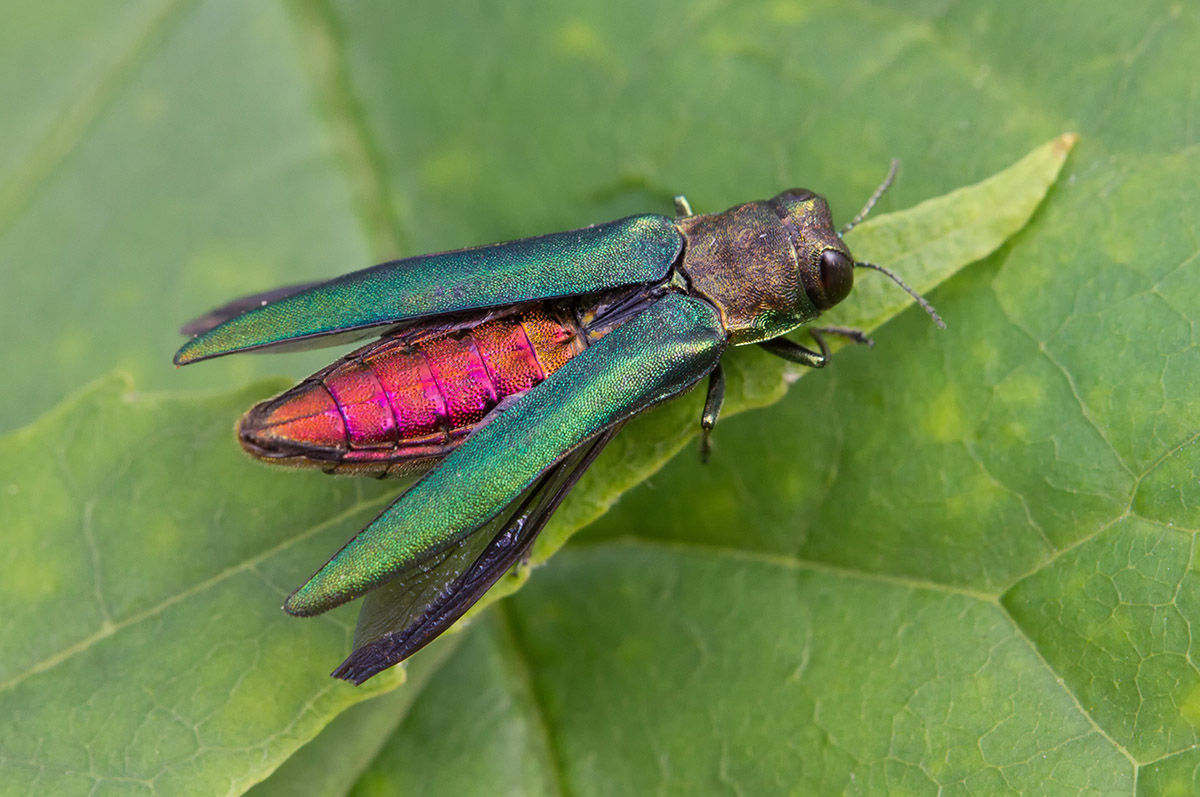This high-resolution, close-up photo captures an emerald ash borer resting on a green leaf, which spans the background of the image. The bug, occupying much of the frame, displays a striking metallic coloration. Its elongated, slender body exhibits a vibrant pink-orange hue beneath its narrow, iridescent wings, which range from a deep emerald green to a lime green towards the tips. A second set of thin, translucent black wings is partially visible beneath the primary ones. The insect's head, a dark deep gray with subtle yellow and green accents, is marked by two large black eyes and antennae. The detailed image, likely intended for scientific study or educational purposes, emphasizes the bug's jeweled, metallic appearance and shows fine details such as its thin metallic legs. The setting features another leaf in the background, adding depth to the overall composition.